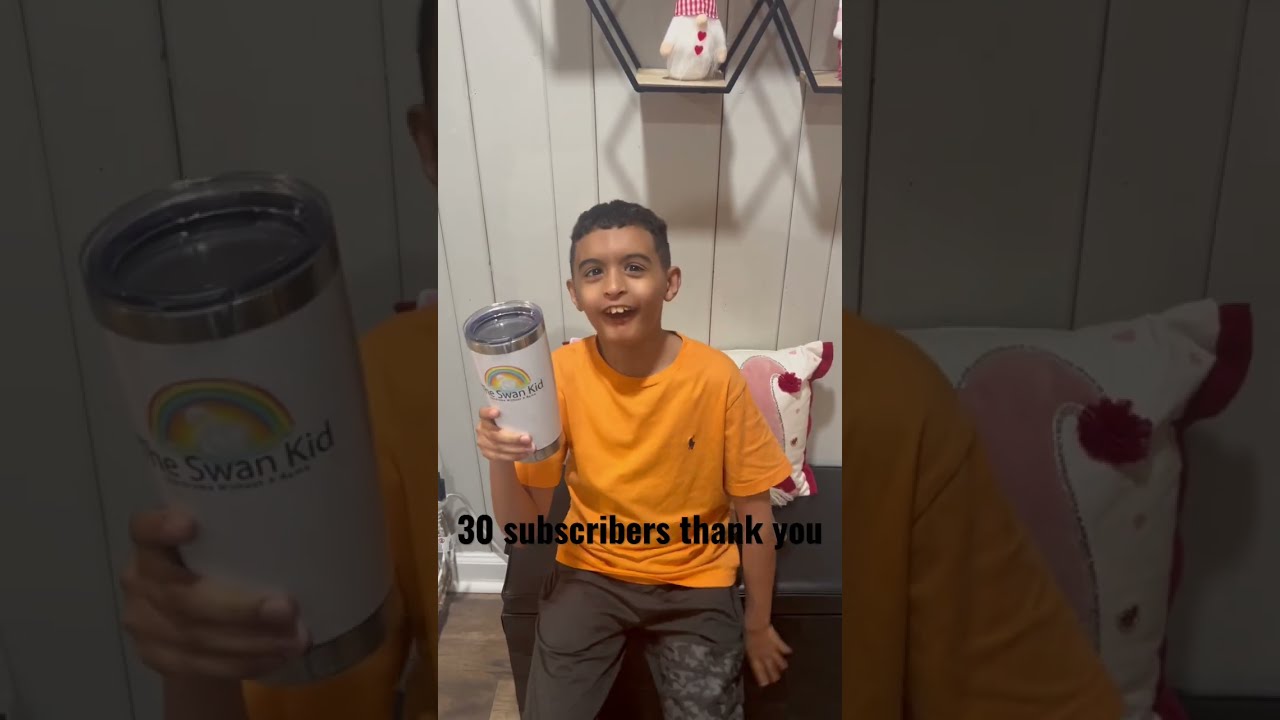The image is a horizontally rectangular composition with darkened sides that frame a central, vertically oriented color photograph. Featured prominently in the center is a young boy, approximately 8 to 10 years old, with dark skin and a beaming smile. He is dressed in an orange T-shirt with the text "30 subscribers, thank you" across the bottom and khaki pants, though some describe them as green trousers. The boy is seated on a black storage bench with a padded leather top, accompanied by a red, pink, and white pillow behind him and a paneled white wall adorned with a geometric shelf holding various Valentine-themed gnomes. 

In his right hand, he holds a white donation jar that features a rainbow design and the words "SWAN KID." The boy radiates excitement and joy. Flanking the central photograph, the background comprises the same photograph zoomed in and darkened, providing a close-up view of the jar on the left, though obscured by the dark overlay. The overall quality of the image is medium, and its style is photographic and representational, similar to social media content.